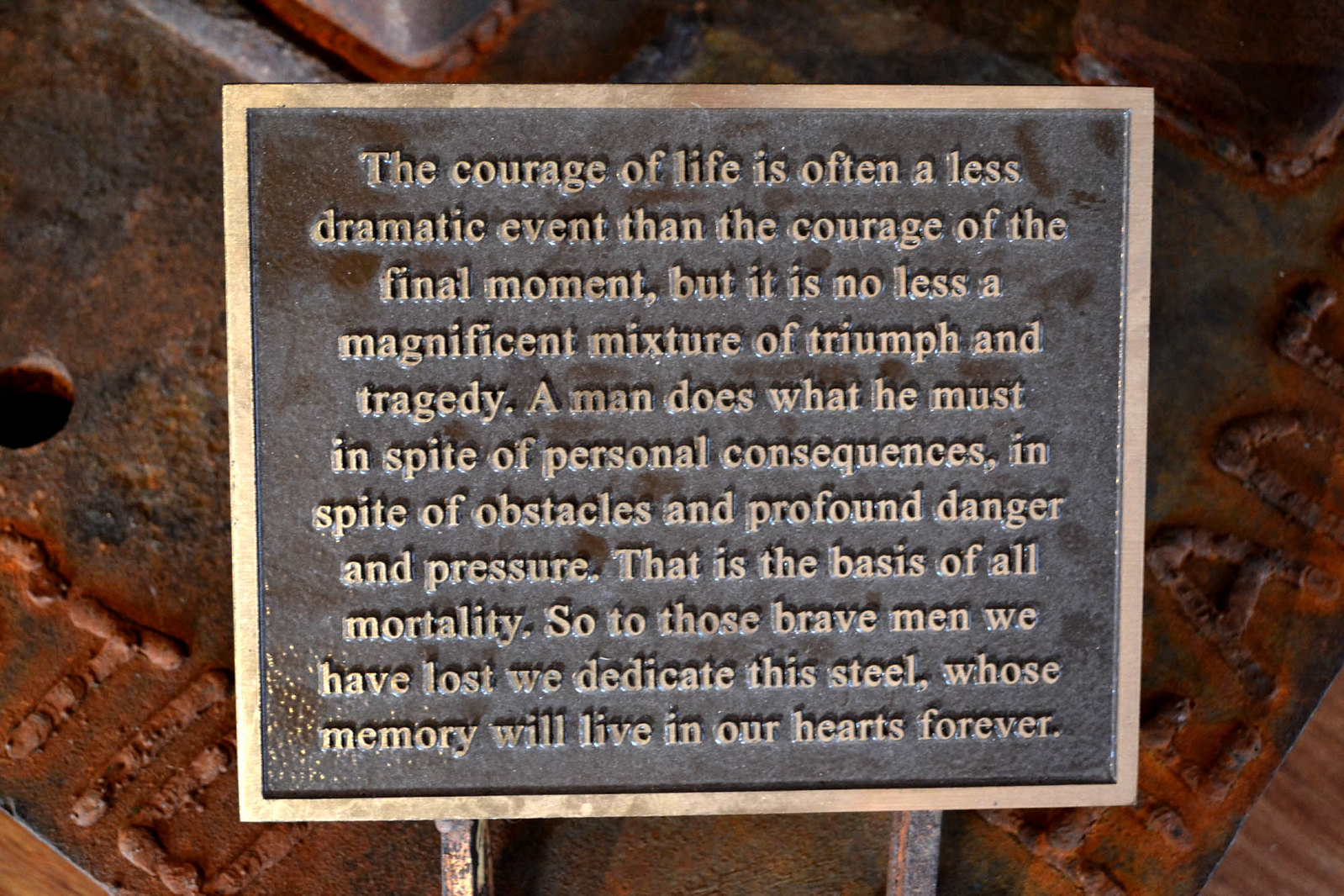The image showcases a plaque encased in a gold frame against a dark brown background with rust-like markings. Central to the plaque is a copper-colored square featuring a metallic inscription that reads: "The courage of life is often a less dramatic event than the courage of the final moment, but it is no less a magnificent mixture of triumph and tragedy. A man does what he must in spite of personal consequences, in spite of obstacles and profound danger and pressure. That is the basis of all morality. To those brave men we have lost, we dedicate this steel whose memory will live in our hearts forever." This plaque, possibly found at the base of a war memorial or a statue honoring fallen soldiers, stands out against the rusty, textured wall behind it.